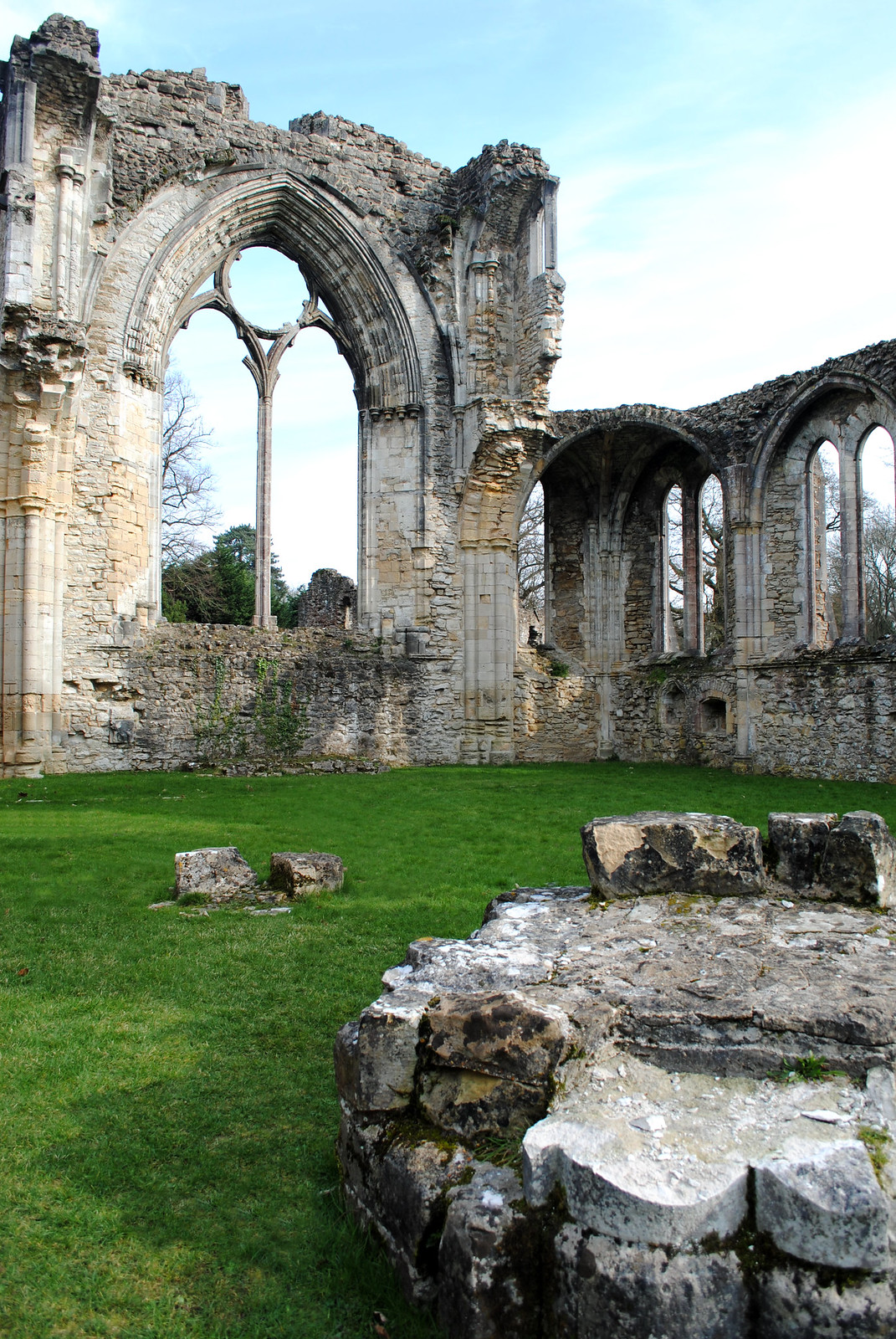This photograph captures the serene and haunting beauty of an ancient courtyard in ruins, likely the remnants of a church or cathedral. Dominating the foreground, there is a large stone table adorned with several square-shaped stones. The lush green grass carpets the courtyard, contrasting with the timeworn stone structures. Scattered across the grassy expanse, two large, loose stones lead the eye towards the more prominent architectural elements. 

At the heart of the image stands a towering wall, featuring splendid cathedral-style architecture. Though the windows are now mere open arches, their intricate design with circular and arched forms still captivates. A passageway with classic arched windows connects different parts of the structure, indicating a higher segment interconnected with a lower one. Behind this wall, the backdrop includes several trees, some with foliage and others bare. 

The stones vary in color from white and tan to shades of gray, adding texture to the scene. The absence of a roof allows natural light to pour in, illuminating the setting and emphasizing the sense of timeless grandeur. This outdoor photograph, likely taken at midday, eloquently captures the essence of historic decay and architectural splendor.